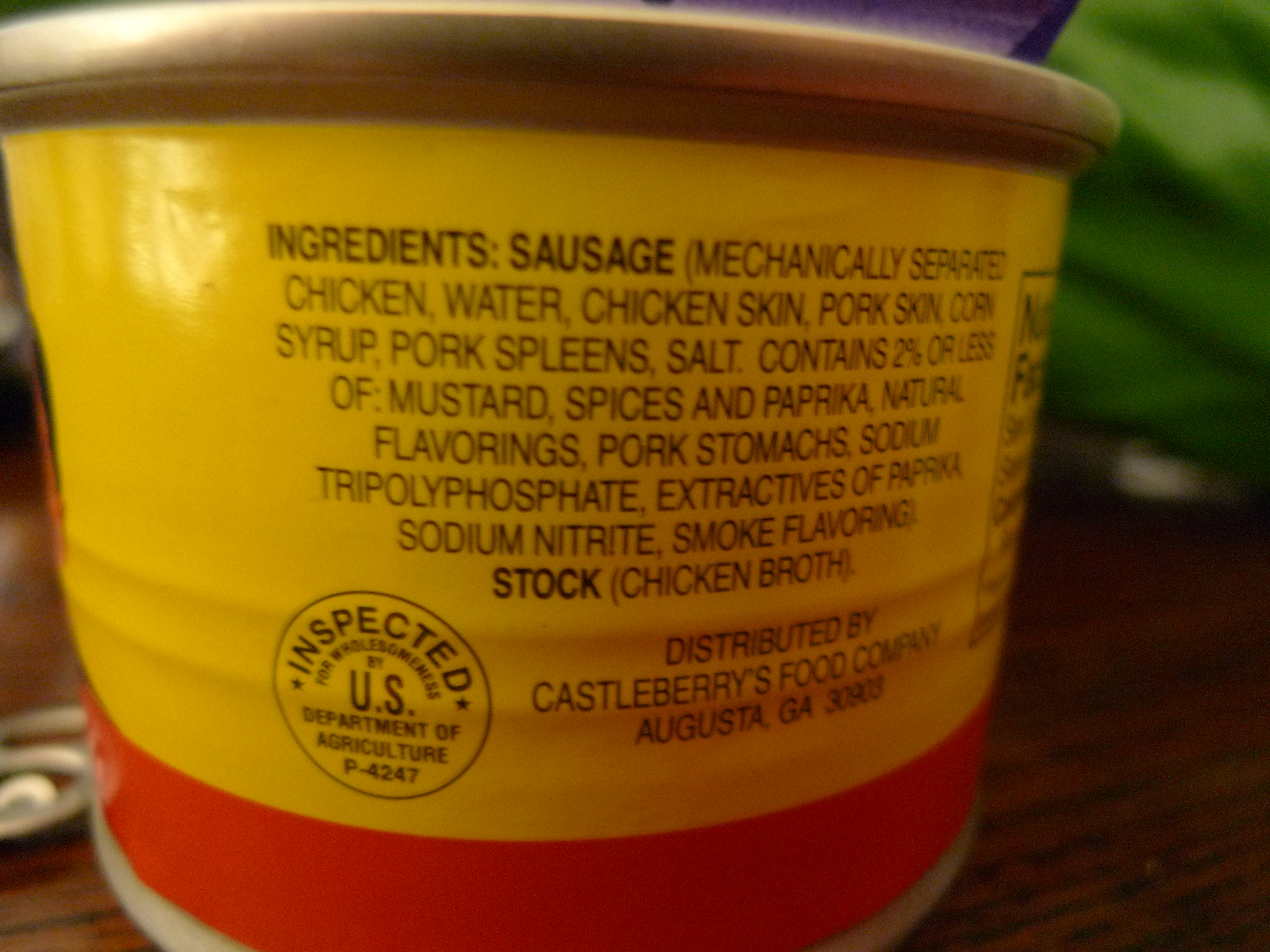The indoor close-up photograph showcases a can of food placed on a dark-grained wooden table with distinctive black stripes, predominantly brown in color. The background features indistinct objects in shades of purple and green, whose details are unclear. Central to the image is the can adorned with a yellow and red label. The label prominently displays an extensive ingredients list including sausage, mechanically separated chicken, water, chicken skin, pork skin, corn syrup, pork spleens, salt, an assortment of spices such as mustard and paprika, natural flavorings, pork stomachs, sodium tripolyphosphate, extractives of paprika, sodium nitrate, smoke flavoring, stock, and chicken broth. It states the product is distributed by Castleberry's Food Company, Augusta, Georgia, and bears a USDA inspected label, signaling its compliance with food safety standards.